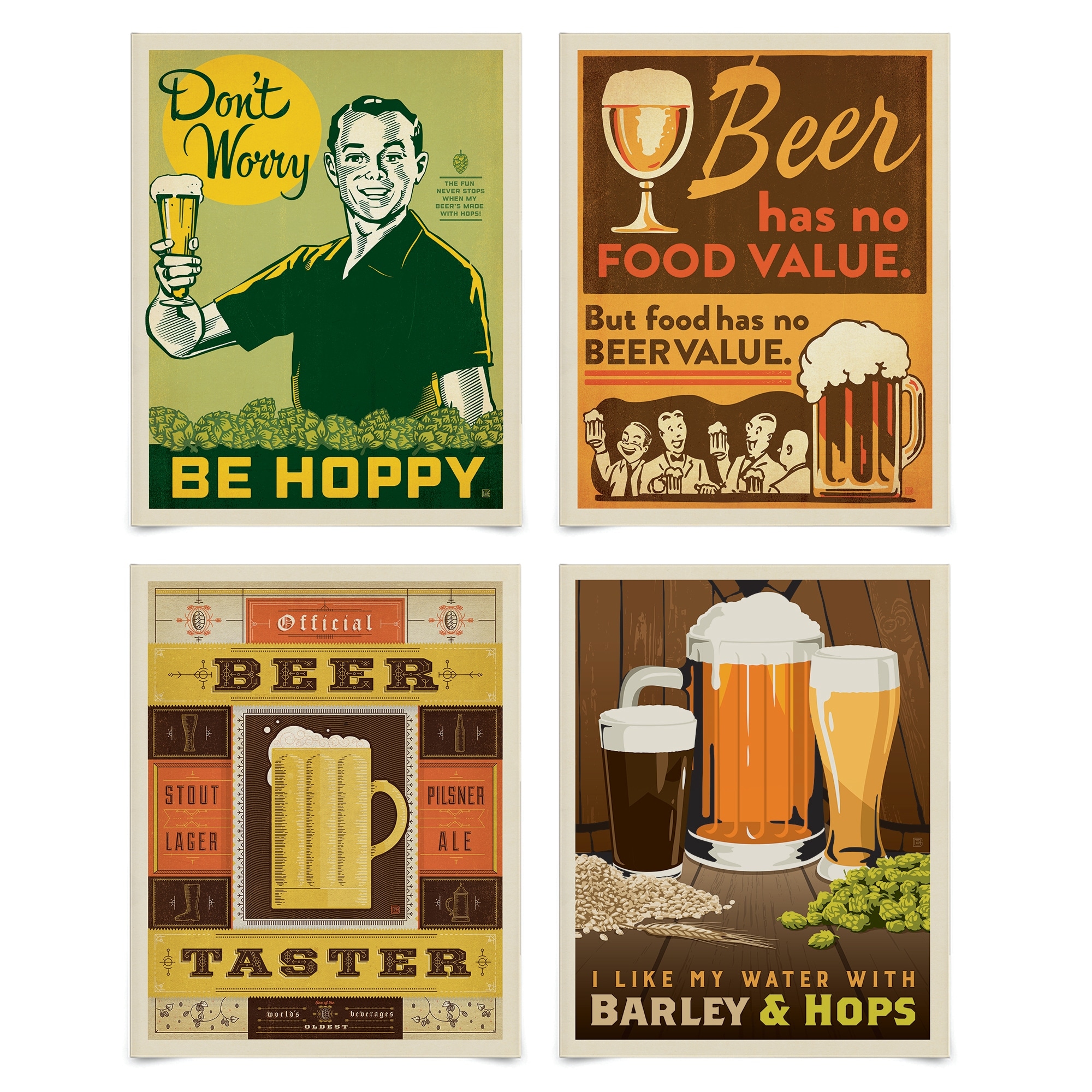This image showcases four distinct vintage-style posters, each bordered by a light gray frame and arranged on a white background, intended for product commercial listings. 

The top left poster features a green background with multiple cartoon beer hops and an animated man visible from the waist up, holding a beer sign with a comically thick forearm. The top left corner reads, "Don't Worry," and the top right says, "Beer has no food value, but food has no beer value." Accompanying the design is the tagline "Be Hoppy" in yellow text at the bottom.

The top right poster combines a brown and yellow backdrop, displaying a beer glass against the brown portion with the heading, "Beer has no food value." Below this, in the yellow section, the same glass accompanies the text, "But food has no beer value," finishing with an image of adults clinking beer glasses.

The bottom left poster has a central image of a beer glass, framed and labeled "Official Beer Taster." Surrounding it are the names "Stout," "Lager," "Pilsner," and "LA," while the background features line drawings of various beer-related items, such as a boat, jar, jug, pitcher, and bottle.

Finally, the bottom right poster depicts a wooden wall and table with an array of beer glasses, grain, and green leaves. A large beer glass dominates the scene with the caption, "I like my water with barley and oats."

Together, these posters create a cohesive and engaging visual presentation for craft beer enthusiasts, highlighting humorous and clever taglines connected through the theme of beer.